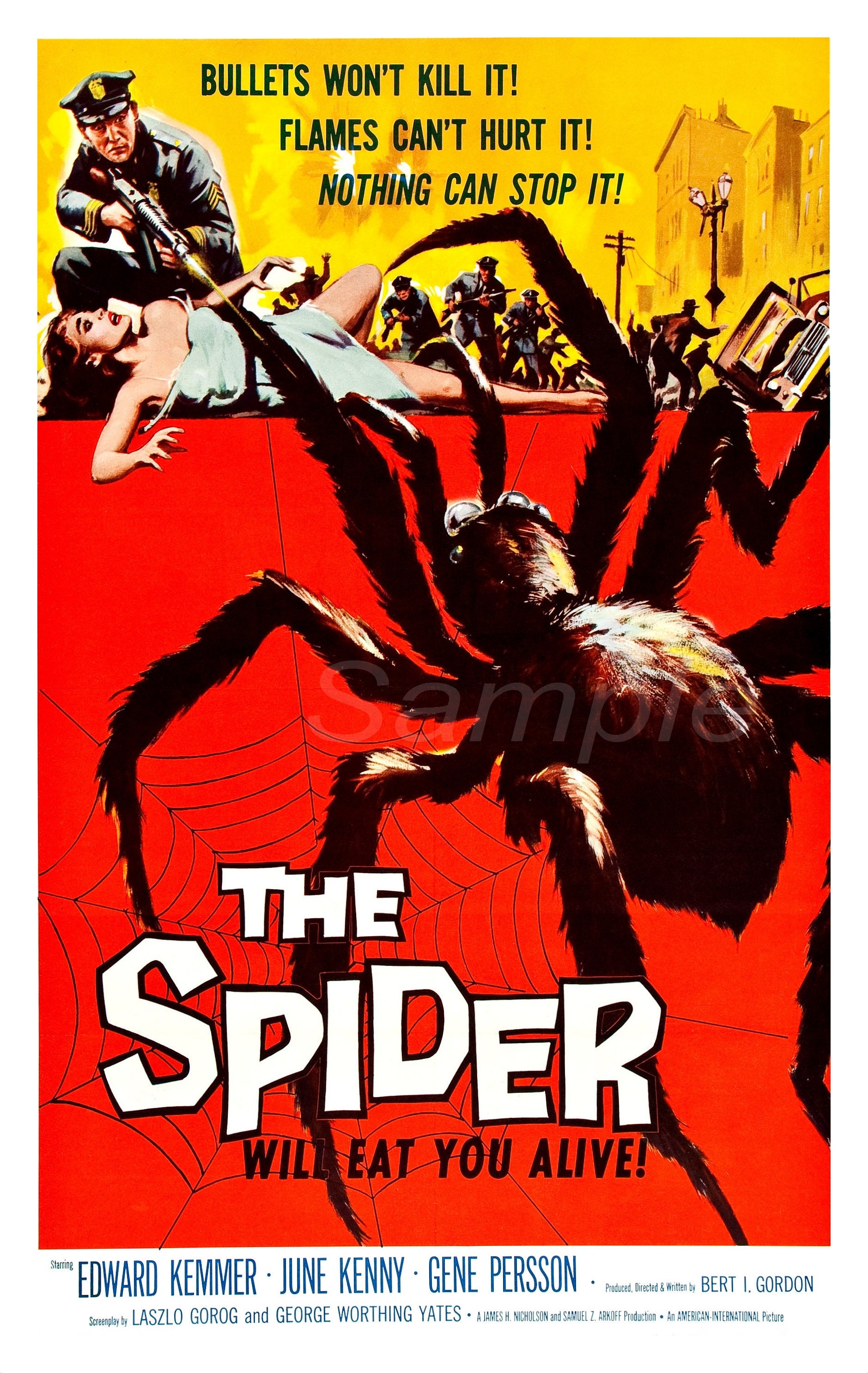A captivating and nostalgic hand-drawn or painted movie poster for "The Spider" captures the surreal terror of a classic creature feature. Dominated by a striking color palette, the upper third of the poster features a golden-hued background adorned with several multi-story buildings, setting a scene of urban chaos. In the middle section, a sense of imminent danger is palpable as a nearly overturned car and panicked police officers wielding rifles scramble to confront the menace. One officer is depicted crouching protectively over a woman in a dress who is prone on the ground, aiming his weapon at the colossal arachnid threat.

The bottom two-thirds of the poster contrasts sharply with a vivid red backdrop, upon which an ominous, large spider web is spread, ensnaring the attention of viewers. A gigantic, menacing spider dominates this web, poised perilously close to the terrified woman. The title, "The Spider," is emblazoned in bold white letters, accompanied by the chilling tagline in smaller black text, "Will Eat You Alive." Below the chaotic scene, the names Edward Kimmer, June Kenny, and Jean Person are prominently displayed, highlighting the film’s cast along with mentions of additional key contributors, though the release date is notably absent. This vintage artwork brilliantly encapsulates the thrilling essence of the movie, promising a spine-chilling viewing experience.